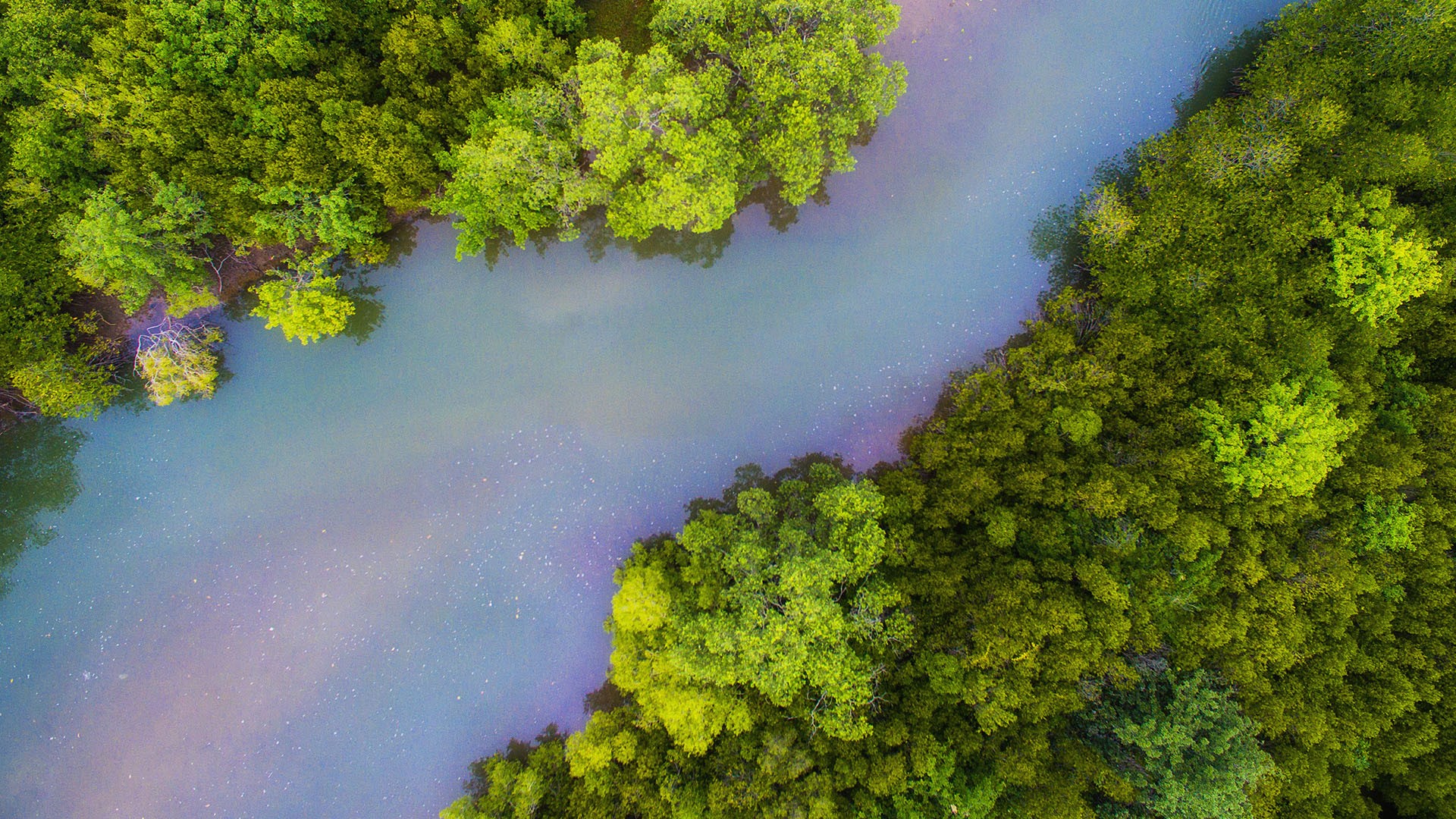This image is a bird's eye view of a river that flows diagonally from the bottom left corner to the top middle right. The river's surface shimmers with a rainbow-like, sparkly hue that appears almost otherworldly, reminiscent of glitter and purple pixie dust, giving it an unreal, space-like quality. On either side of the river, dense forests flourish with a variety of tree colors and types. The left side features a blend of light yellow-green leaves and dark trees, particularly toward the top left. The right side of the image showcases a similar vibrant mix, with dark green and light green foliage, as well as a hint of purple at the bottom right. These trees, possibly mangroves, extend out over the water, creating a lush, tropical scene that evokes the feel of a swamp or a tropical mangrove forest, much like those found in Florida.